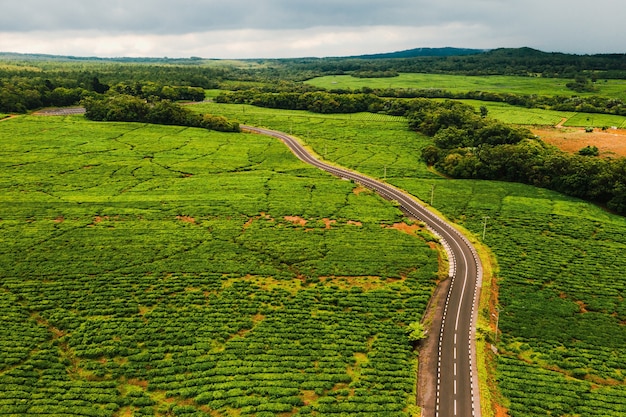The image depicts an aerial view of a scenic countryside landscape under a gray, cloudy sky that transitions from darker to lighter shades. The central feature is a winding, two-lane paved highway that snakes through lush green fields and farmland, marked by dotted and solid white lines. The road stretches from the foreground and weaves its way towards a distant tree line, disappearing into a dense forest area. On either side of the highway, the verdant fields are interspersed with patches of red dirt and areas that look arid and cracked, possibly indicating a need for irrigation. The landscape is dotted with clusters of tall, thick green trees and shrubs, and there are also some areas of bare dirt. Power and phone lines run along one side of the road, along with traffic lights and streetlights. In the background, low rolling hills give way to a distant range of tree-covered mountains or hills, creating a striking backdrop to the scene. The sky overhead is overcast, suggesting an imminent rain.